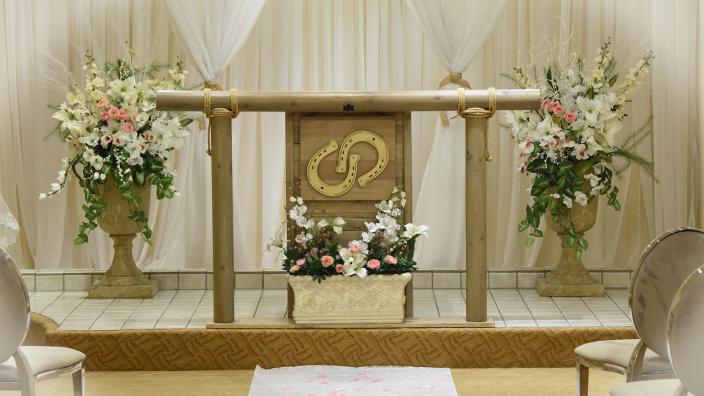The photograph depicts a wedding venue with a small tiled stage at the front. The stage is adorned with bouquets of white and pink flowers placed on stone vases on either side, with a small bouquet positioned centrally in front of the stage. The backdrop of the stage is lined with white curtains, adding a touch of elegance. A wooden hitching post, reminiscent of those used to tether horses, is positioned on the stage, featuring a podium behind it. The podium displays two interlocking horseshoes in a yellow hue, symbolizing good fortune. The seating area consists of cushioned chairs with dark grayish-brown oval backs arranged on either side of a central aisle. This aisle is carpeted in brown with a white fabric strip running down the middle, guiding the way towards the stage. The overall ambiance suggests a serene and intimate setting, perfect for a wedding ceremony.